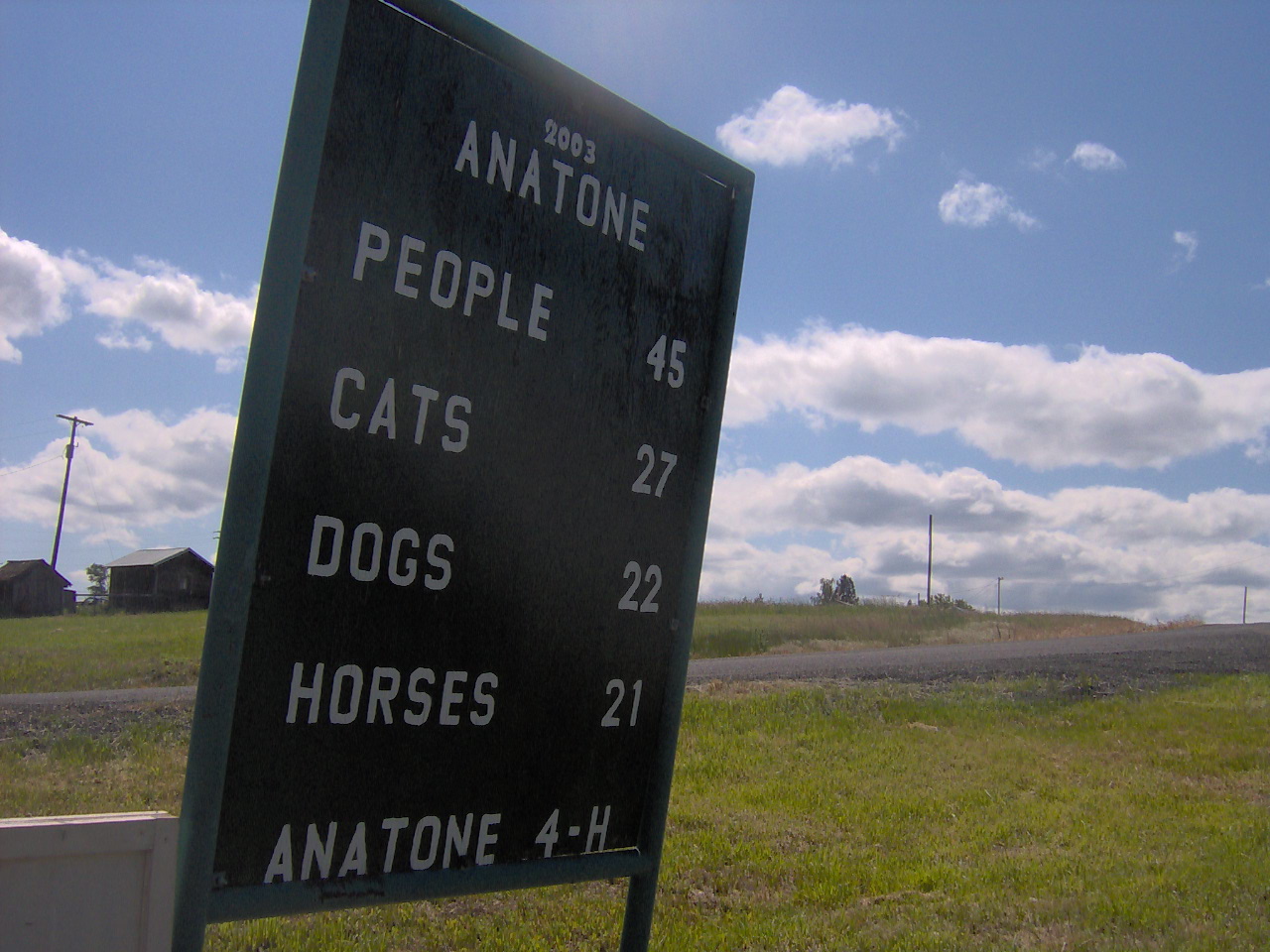The image features a quaint, solitary sign displaying the population statistics for Anatone, a seemingly remote and quiet locale. The sign, framed in green metal with a black background, is the type where white letters can be manually placed. It stands alone against a backdrop of an expansive field with a solitary road meandering by. A small house is visible in the distance behind the field, with power lines stretching overhead. The sky is a light blue canvas adorned with fluffy white clouds. According to the sign, which was put up by the Anatone 4-H Club, Anatone is home to 45 people, 27 cats, 22 dogs, and 21 horses. The whimsical inclusion of pets highlights the charm and close-knit nature of this tiny community.